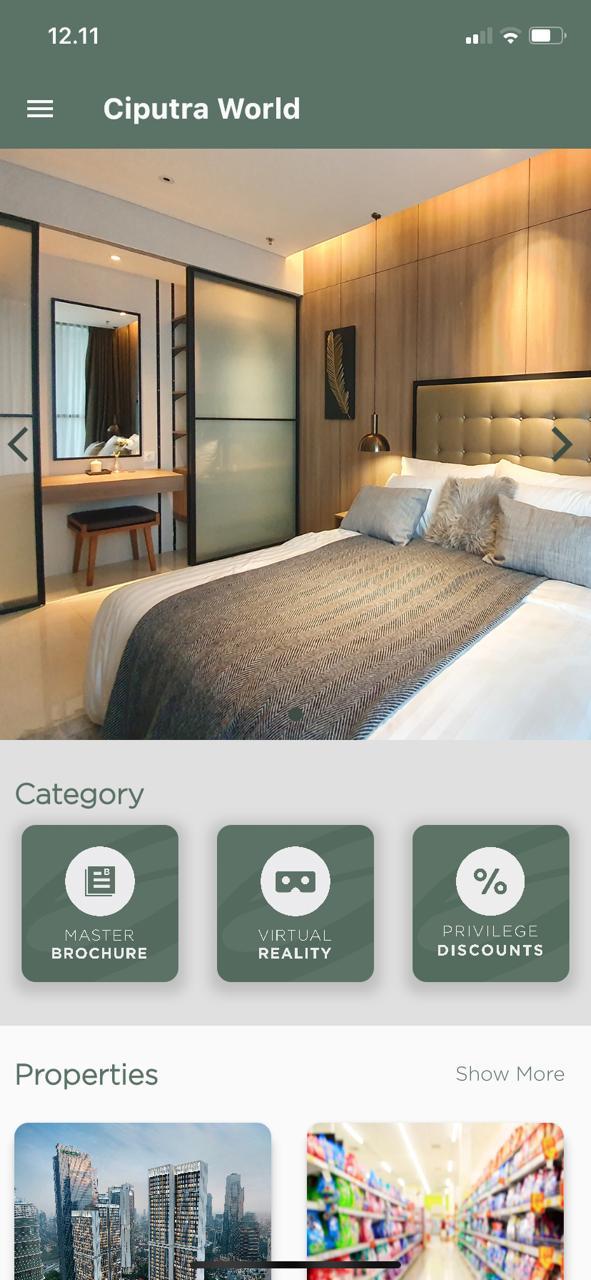This image appears to be a screenshot from the app or website "Seputra World." It features a tastefully designed bedroom, boasting a serene and sophisticated ambiance. The centerpiece is a bed adorned with crisp white linen, a gray blanket, and an assortment of gray and white pillows. A beautifully upholstered headboard complements the wooden wall that is accentuated by elegant drop-down pendant lights.

To one side of the room, there is a semi-opaque, glass-like door, which, due to its blurriness, could either be a cupboard or a shower. Centrally located on the wall is a mirror, positioned above a wooden bar that functions as a vanity table. On the opposite side, another door or glass-like window can be seen, adding to the room's airy feel.

At the bottom of the screenshot, several tabs read: "category," "master," "brochure," "virtual reality," "privilege," and "discount." Additionally, it says "properties" with an option to "show more." The lower portion of the screenshot includes two small images: one depicting a cityscape, and the other showing an aisle in a store.